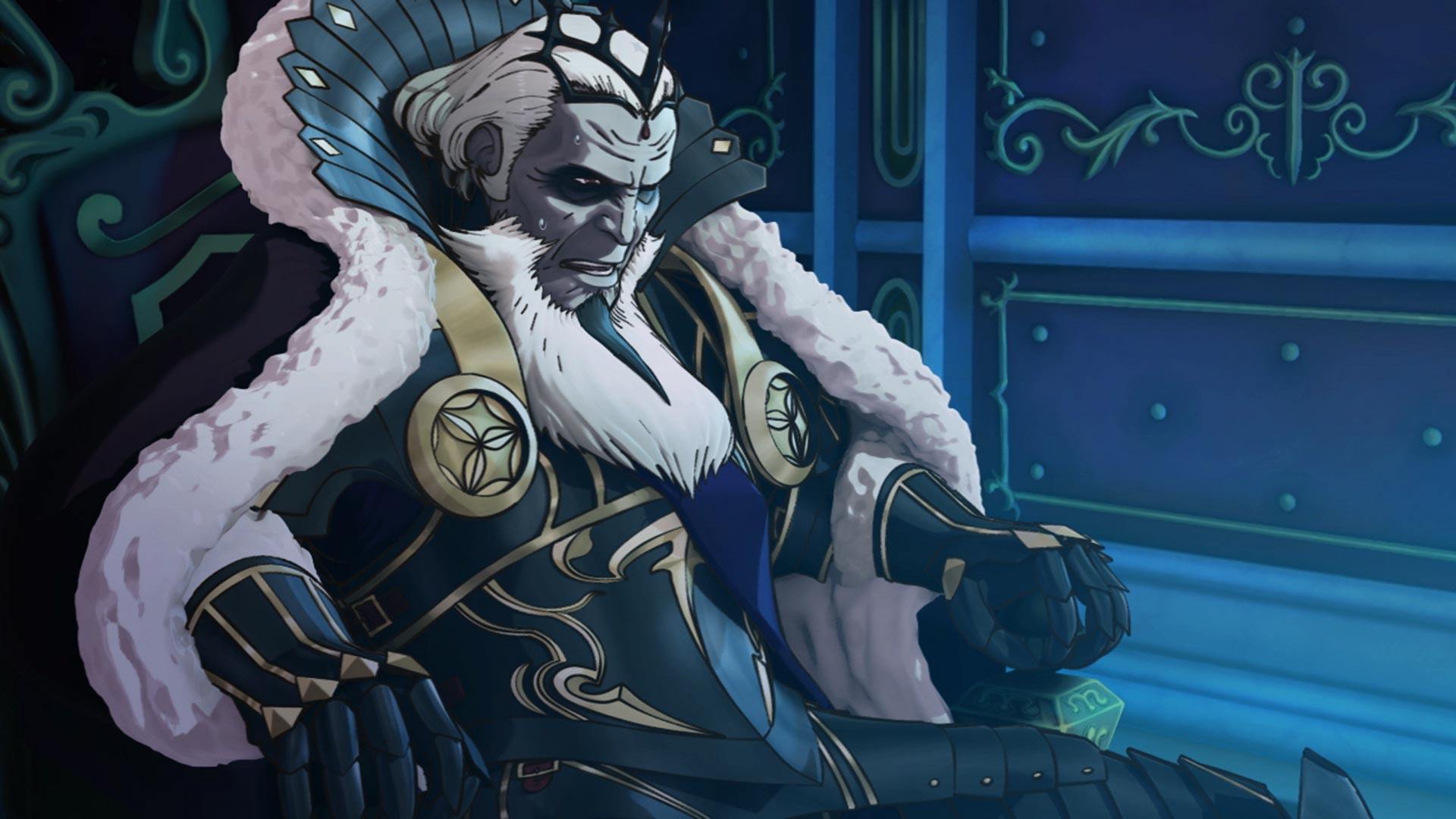This color illustration, in a comic book style with a landscape orientation, features an imperial, possibly villainous character seated slightly off-centered in an ornate chair. The character, reminiscent of an anime or cartoon figure, has a striking appearance with long white hair, a long white beard with a pointed black section, and a scowling expression. He dons heavy eye makeup with blue eyeliner. His outfit is elaborate, including a crown made of black antlers and a grand stand-up collar of black plastic in a fan shape, complemented by a surrounding arc of white fur lining his robe. His attire consists of a pink fur-trimmed jacket with a hood, dark blue armor adorned with golden motifs, circle-shaped metal clasps on the shoulder straps, and black gloves. The armor has a brass-like finish with rivets on the legs and chest. The character sits in a chair positioned towards the left side of the image while behind him, a section of the wall upholstered in dark blue with golden insignia designs and white trim can be observed. The colors within the image, including purple, gray, white, green, gold, and black, enhance the intricate and regal yet somewhat dark aesthetic.